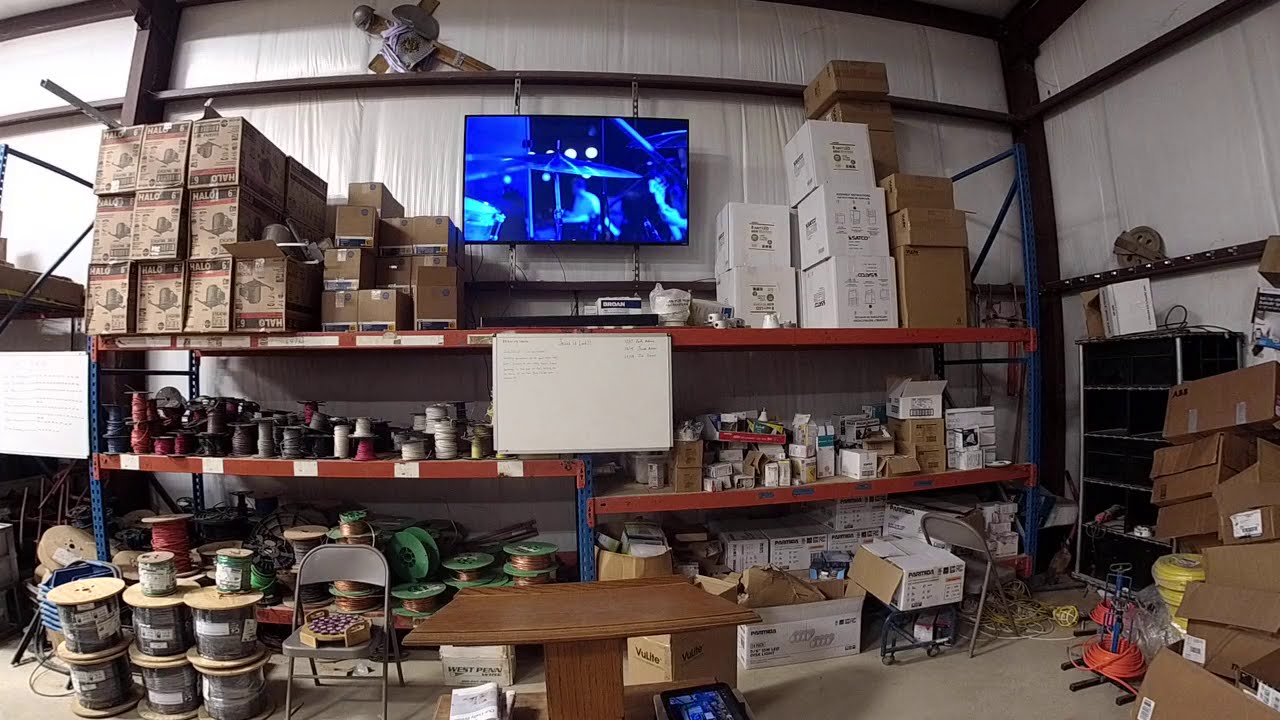The image depicts an industrial storage area characterized by white walls with black framing. Central to the scene is a shelving unit with a blue frame and orange shelves, used to store various items. The top shelf holds an assortment of brown and white cardboard boxes. Mounted on the wall in the center is a flat-screen television, which is on and appears to be displaying a band playing. Below this on the second shelf, there are several spools of wire, with additional cardboard boxes placed to the right. The very bottom shelves are occupied by more spools of copper wire and additional white cardboard boxes. In the lower center of the image is a short wooden table with several cardboard boxes at its base. To the right, another black shelving unit is partially visible against the wall, also laden with boxes that vary in appearance. The area overall is filled with a variety of items, giving it a cluttered but organized feel.